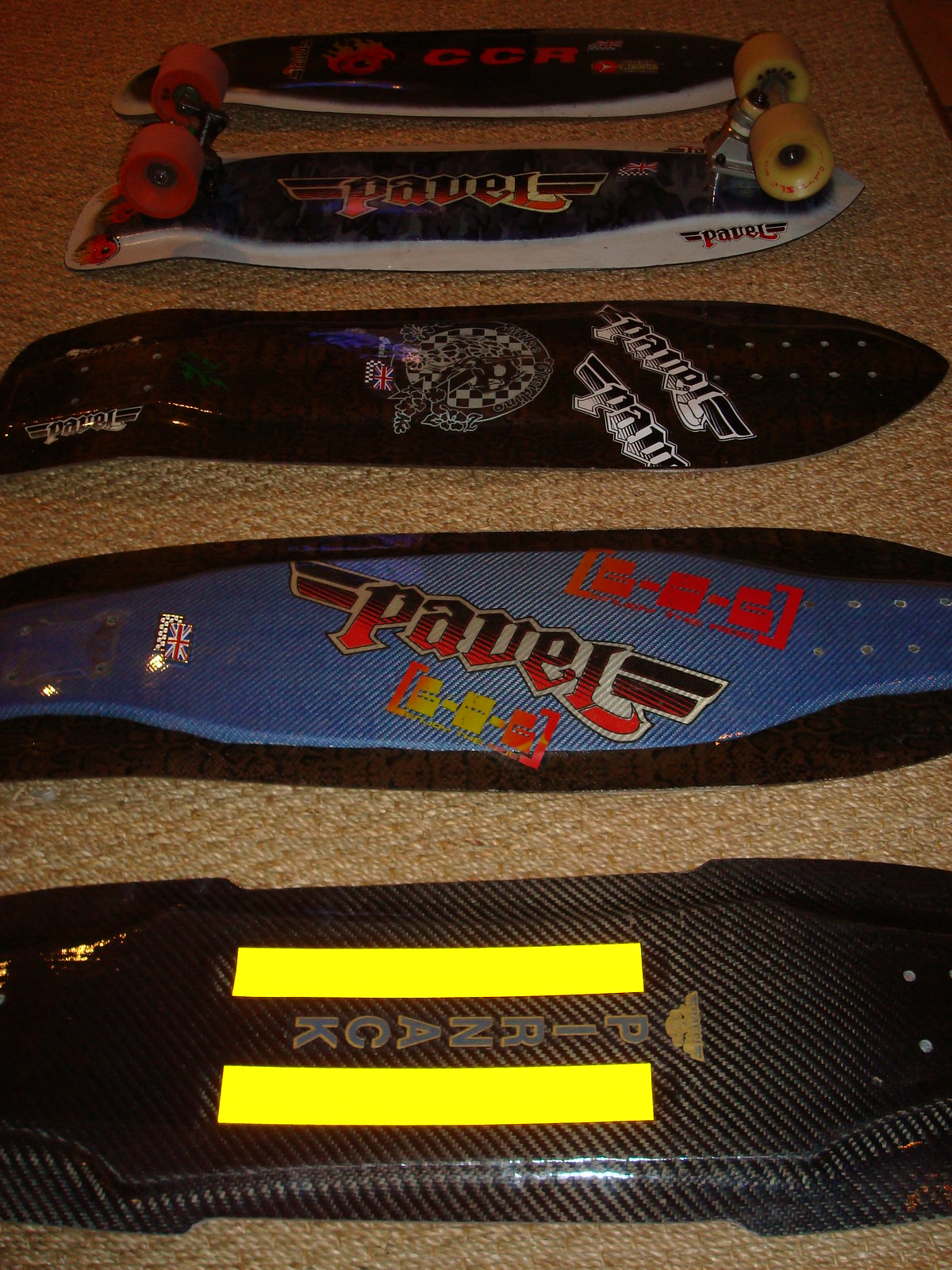This vertically-oriented color snapshot captures five skateboards lined up from the bottom to the top of the image, positioned on a beige textured surface, likely a carpet. The skateboards display a variety of colors and detailed designs with text. The first skateboard at the bottom is black with two neon yellow stripes and prominently shows the text "PIRNACK." The second skateboard, which is blue with red and yellow designs, features the text "Pavel" in red. The third skateboard, predominantly black with white and black designs and a hint of purple, also includes the text "Pavel." The fourth skateboard, the only one equipped with wheels, is black with red and yellow designs, showing the text "Pavel" and encircled by a white rim; its wheels are mismatched, with yellow on the right and orange on the left. The fifth and final skateboard is black with a white rim and displays the text "CCR" in orange. The image is taken under artificial lighting and slightly underexposed, giving it a warm yellow tint.